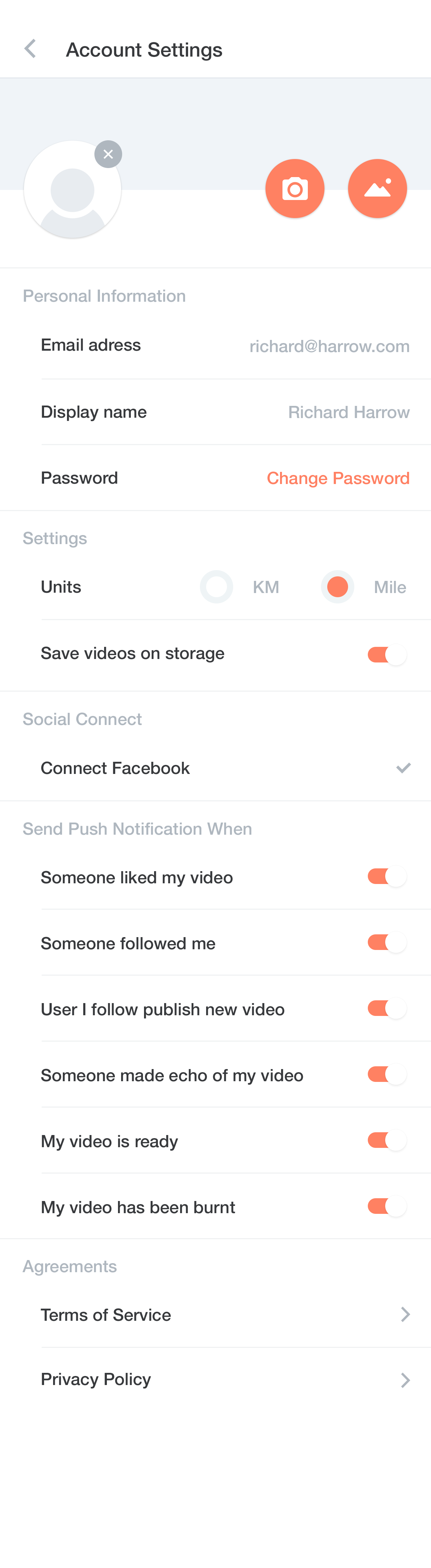**Detailed Caption for a Screenshot of Mobile Phone Settings:**

The image is a screenshot of the "Account Settings" page on a mobile phone, featuring a clean and intuitive layout with a white background. 

- **Header Section:**
  - The top left corner clearly displays the title "Account Settings" in a bold black font.

- **Profile Section:**
  - Directly below the header, there is a large gray rectangle. On its left side, a white circle contains a gray silhouette of a human figure. A smaller gray circle with a white "X" in its upper right corner suggests a pending action or removal.
  - To the right of this circle, two red icons stand out—a camera icon and an icon depicting a mountain with a sun, indicating options to upload or change the profile picture.

- **Personal Information:**
  - Below the profile section, there is a gray dividing line. The text "Personal Information" is written in gray font.
  - Listed under this heading are:
    - **Email Address:** "richard@harrow.com"
    - **Display Name:** "Richard Harrow"
    - **Password:** The option "change password" is available.

- **Preferences and Settings:**
  - The section labeled "Settings" provides options for unit preferences, with "km" and "mile" available, and "mile" selected.
  - An option labeled "Save videos on storage" shows a toggle switch turned on.

- **Social Connect:**
  - Under "Social Connect," "Connect Facebook" is selected, as indicated by a checkmark.

- **Notifications:**
  - The section "Send push notification when" lists various events, all of which have their respective toggles switched on. These notifications include:
    - Someone liked my video.
    - Someone followed me.
    - User I follow publishes new video.
    - Someone made an echo of my video.
    - My video is ready.
    - My video has been burned.

- **Legal Information:**
  - At the bottom, links to "Agreements and Terms of Service" and "Privacy Policy" are provided.

This structured view ensures that users can easily navigate and manage their account settings, personal information, preferences, social connections, notifications, and legal acknowledgments.